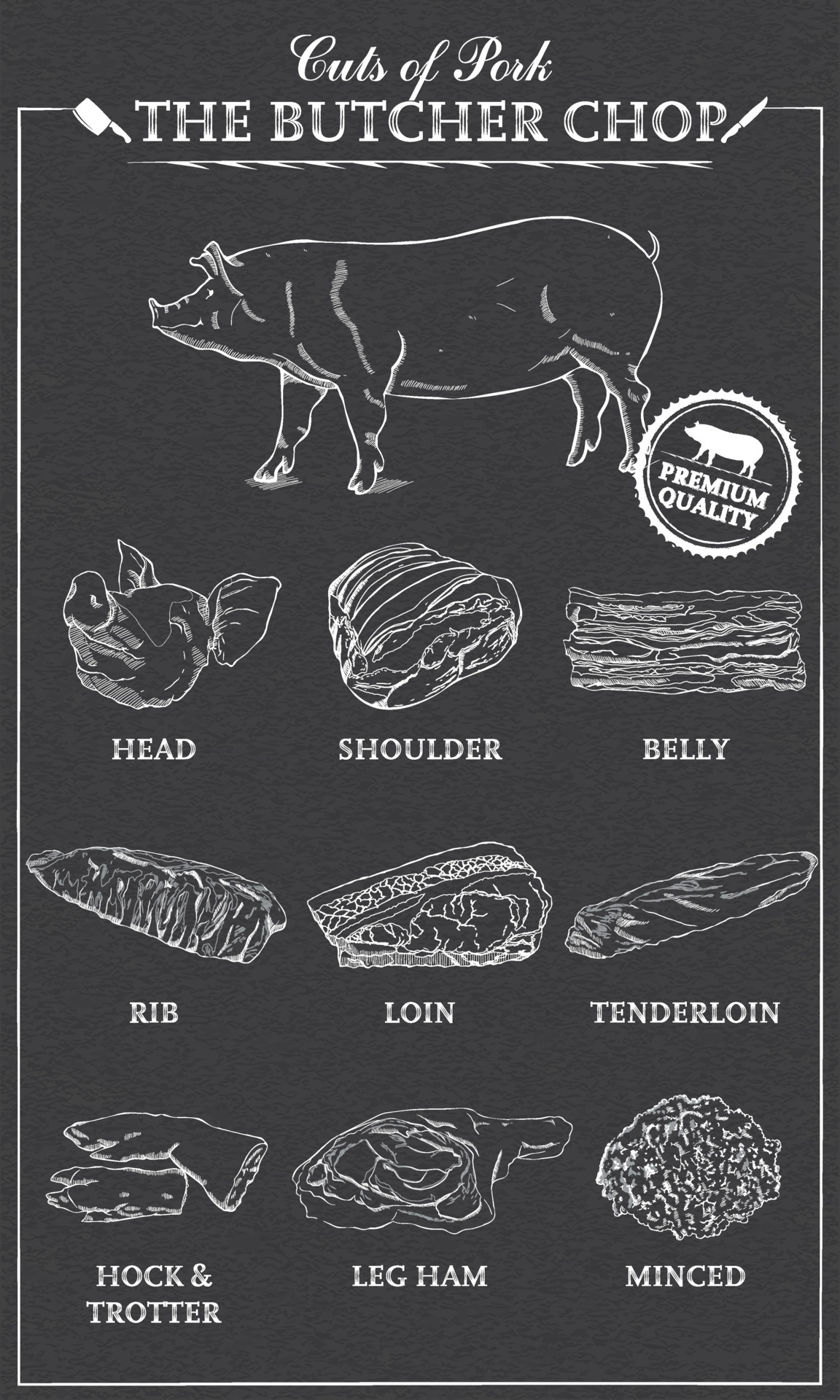This is a detailed black and white butcher shop poster with a dark gray background, titled "Cuts of Pork" in cursive, followed by "The Butcher Shop." Overlaying the top left corner is a meat cleaver, and a knife adorns the top right, creating a balanced visual appeal with a thin white border extending around the edges of the entire poster. The center features a detailed chalk-like outline of a pig, segmented to illustrate nine specific cuts of pork: head, shoulder, belly, rib, loin, tenderloin, hock and trotter (depicting the feet), leg ham, and minced. To the right of the pig is a seal marked "Premium Quality," emphasizing the quality of the shop’s offerings. This poster perfectly blends an instructional guide with rustic butcher shop aesthetics.